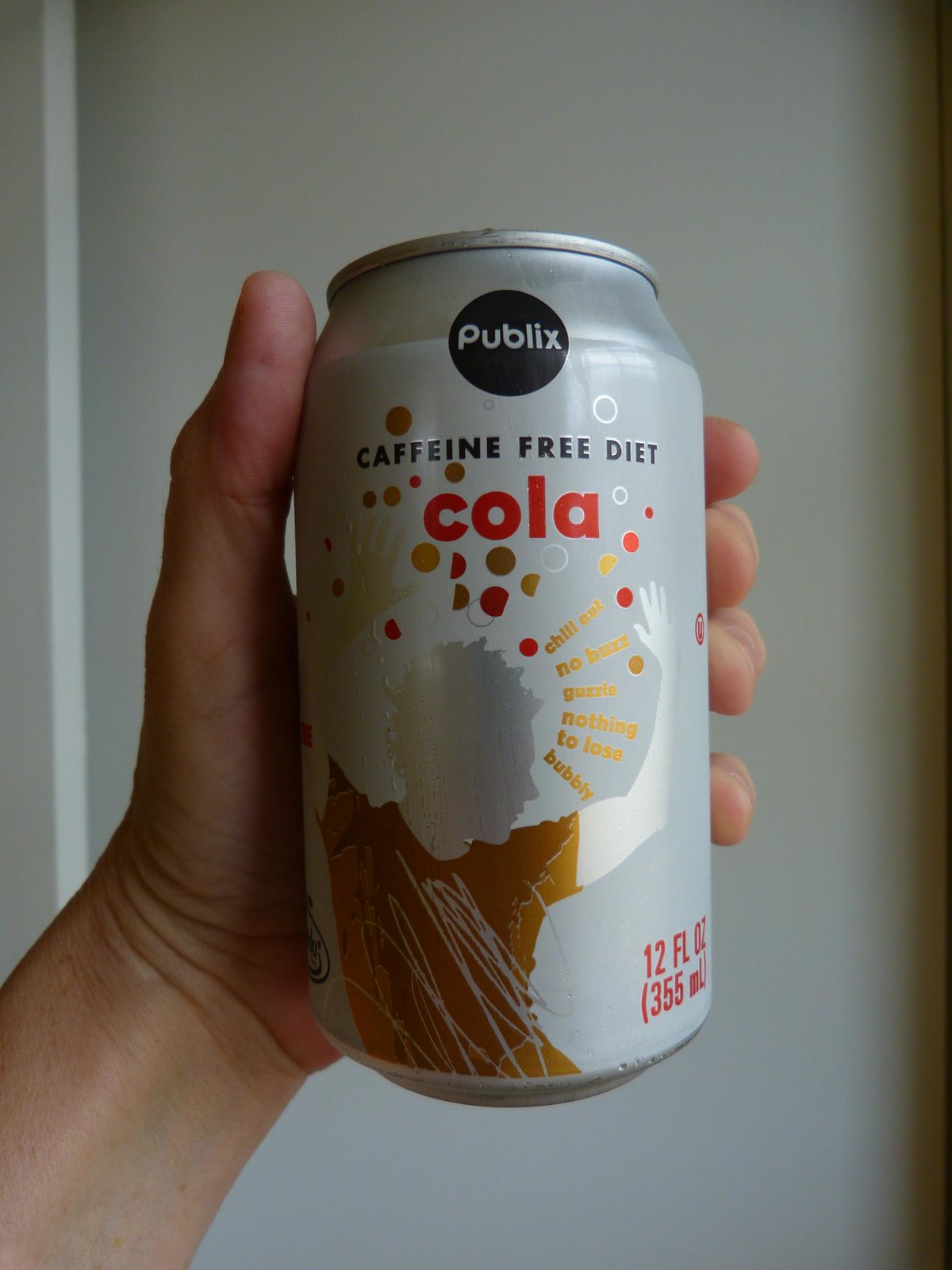This image captures a 12 fluid ounce (355 milliliters) can of soda from Publix. The can is prominently silver in color and features a striking design. The labeling on the can indicates it is a "Caffeine-Free Diet Cola." The can's visual motif includes an illustration of a man, possibly dressed in a brown shirt, with his arms raised in a jubilant pose, suggesting he might be dancing. Overlaid on this image are the words, "Chill Out, No Buzz, Guzzle, Nothing to Lose, Bubbly." The person holding the can appears to be a Caucasian man, as discerned from the visible hand.